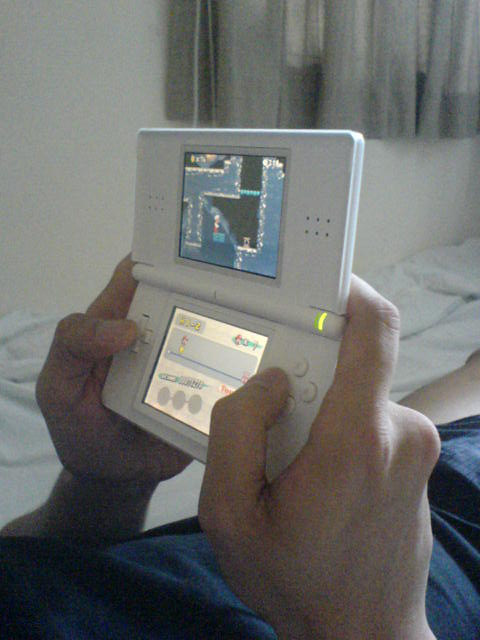This color photograph captures a man reclining on a bed with white bed sheets, partially showing his thigh. He is dressed in midnight blue shorts and a matching blue t-shirt. The man holds a white portable video game console with both hands, each thumb resting on a control button, indicating he is actively playing a game. The console features two screens; the top screen is visibly displaying a game with light blue and dark blue colors and figurine graphics, while the bottom screen holds a different part of the game interface. The console also has control buttons and a joystick mechanism. The background reveals an off-white wall and a partial view of a window draped with sheer gray curtains. Details like six speaker holes around one of the screens suggest that the console provides audible game sounds.